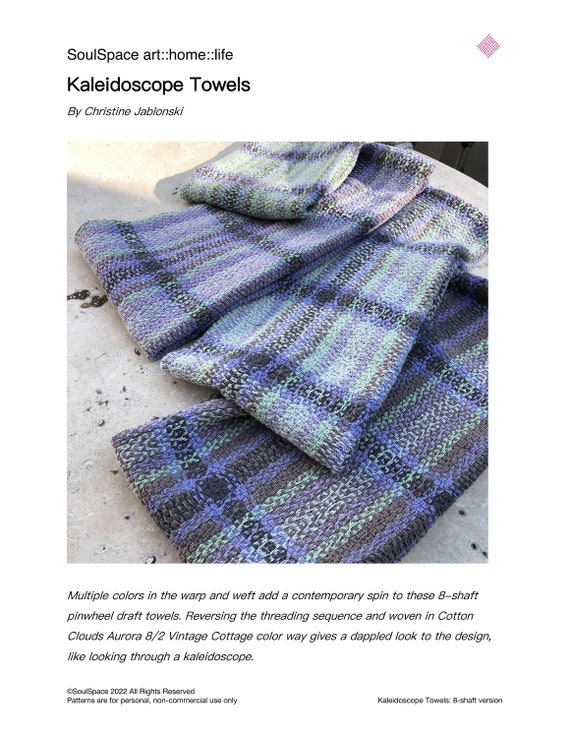This image appears to be a screenshot from a website or social media post advertising a brand of towels named "Kaleidoscope Towels" by Christine Jablonski. At the top left, the text reads "Sol Space: Art :: Home :: Life." The towel, which may also resemble a scarf, is depicted in a plaid pattern composed of light blue, teal, lavender, black, darker gray, and white. The description emphasizes the towel's unique design, noting that the multiple colors in the warp and weft create a contemporary spin on an eight-shaft pinwheel draft, providing a vintage cottage feel. This kaleidoscopic effect gives the fabric a dappled look, reminiscent of viewing through a kaleidoscope.